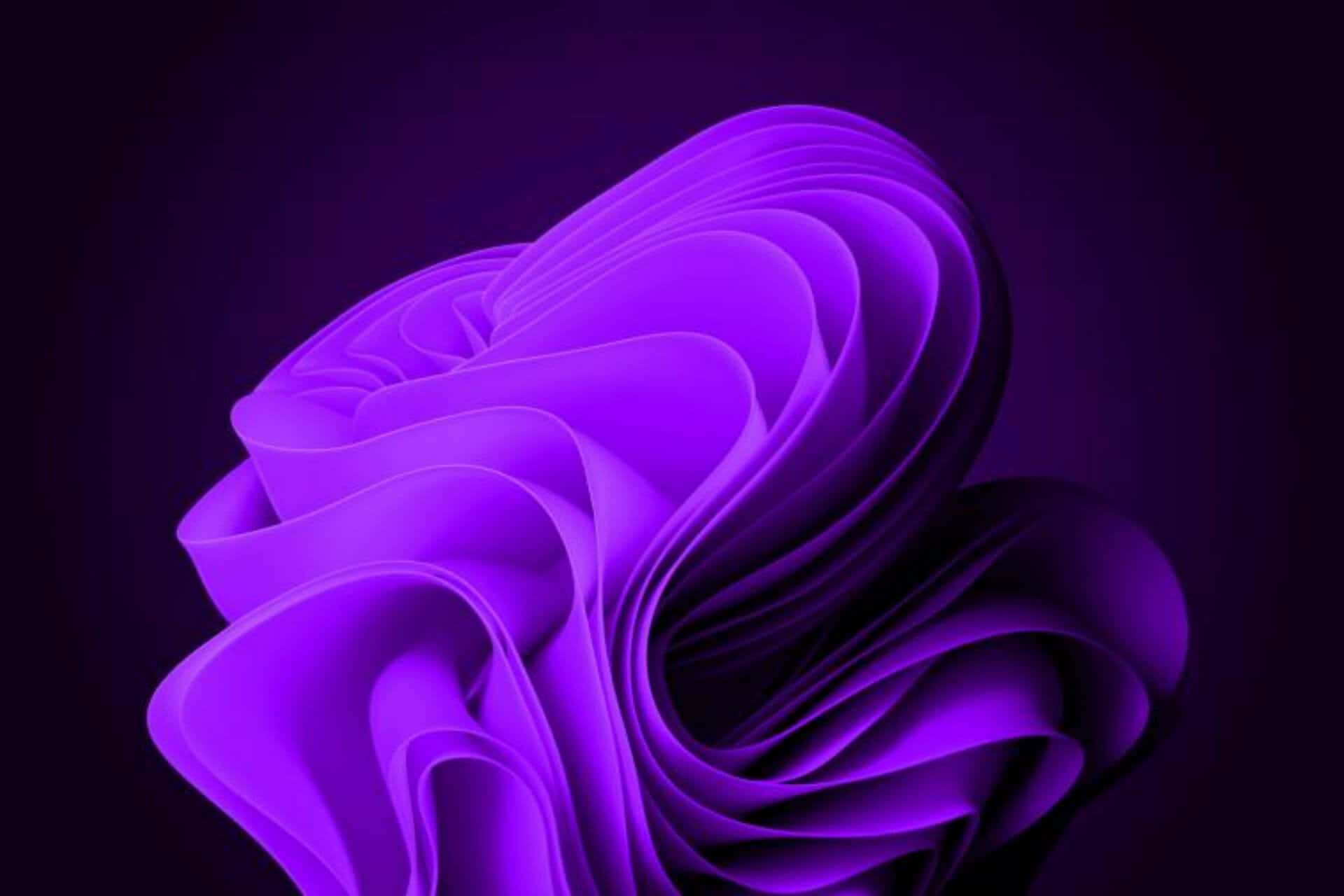The image appears to be a digitally generated square composition with no border. It features a dynamic, multi-layered arrangement of what looks like wavy sheets of fabric or paper, predominantly in varying shades of purple. The background is a dark purple to black gradient that transitions to lighter purple as it moves toward the center, giving the image a subtle glow that emanates outward. The folds and twists of the purple material create a complex, almost floral pattern, reminiscent of petals swirling and cascading in different directions. The left side of the arrangement is illuminated, providing a stark contrast to the darker, crevice-like shadows on the right. The edges of the fabric or paper have a lighter hue, adding to the intricacy and depth of the design. There are no people, animals, or text in the image, making the focus entirely on the abstract, artistic display of light, color, and form.